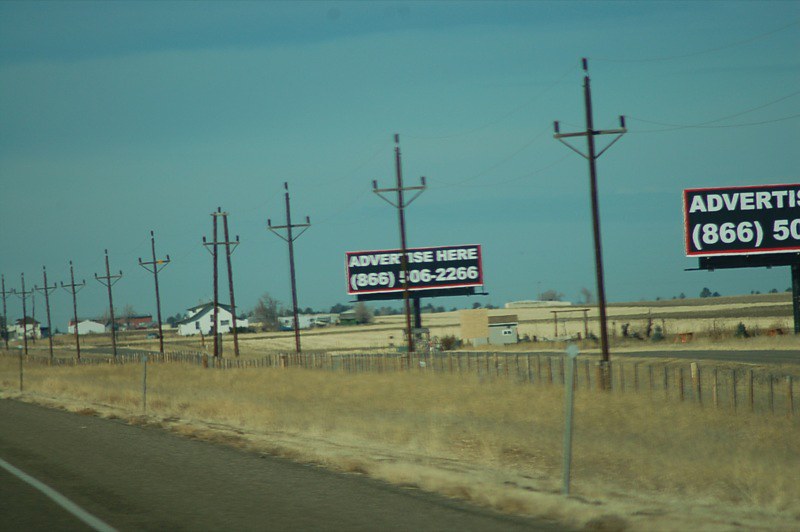The image depicts a rural scene on a sunny day with a medium to dark blue sky adorned with wispy white clouds. On the right side of a black roadway with a distinctive white strip lies a large grassy area where the grass appears dead and brown. Bordering this area is a row of approximately ten power poles, each connected by power lines, alongside a silver or white fence that demarcates what seems to be a farm or ranch. Along this roadside stand two billboards: the nearest one is partially cut off, reading “advertise, 86650,” while the other is fully visible, displaying “advertise here, 866-506-2266.” In the background, white farmhouses with roofs can be seen, completing the picturesque rural setting.